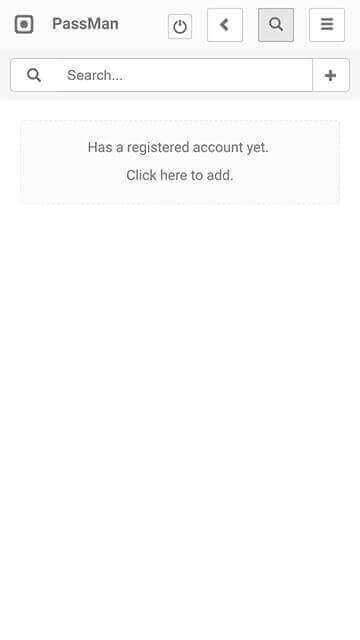The image depicts the interface of the PassMan application. Located at the very top left is the name "PassMan" written in dark grayish text. To the left of the name, there is a square icon enclosing a circle, also in a dark gray hue. Centered at the top of the image is a white square containing a power symbol, indicating a power-on function. Immediately to its right, another white square features a left-pointing arrow. Next to this, a square with a light grayish background holds a darker gray magnifying glass icon. At the top right of the image, the final square with a white background displays three horizontal bars stacked atop one another.

Below these icons, a search bar spans across the screen, designed as a horizontal rectangle. Inside this search bar, on the left side, is a magnifying glass icon followed by the text "search..." On the far right of the search bar, a plus (+) symbol is visible. Beneath the search bar, there's a smaller rectangular section with the instruction, "Has a registered account yet? Click here to add," set against a grayish background.